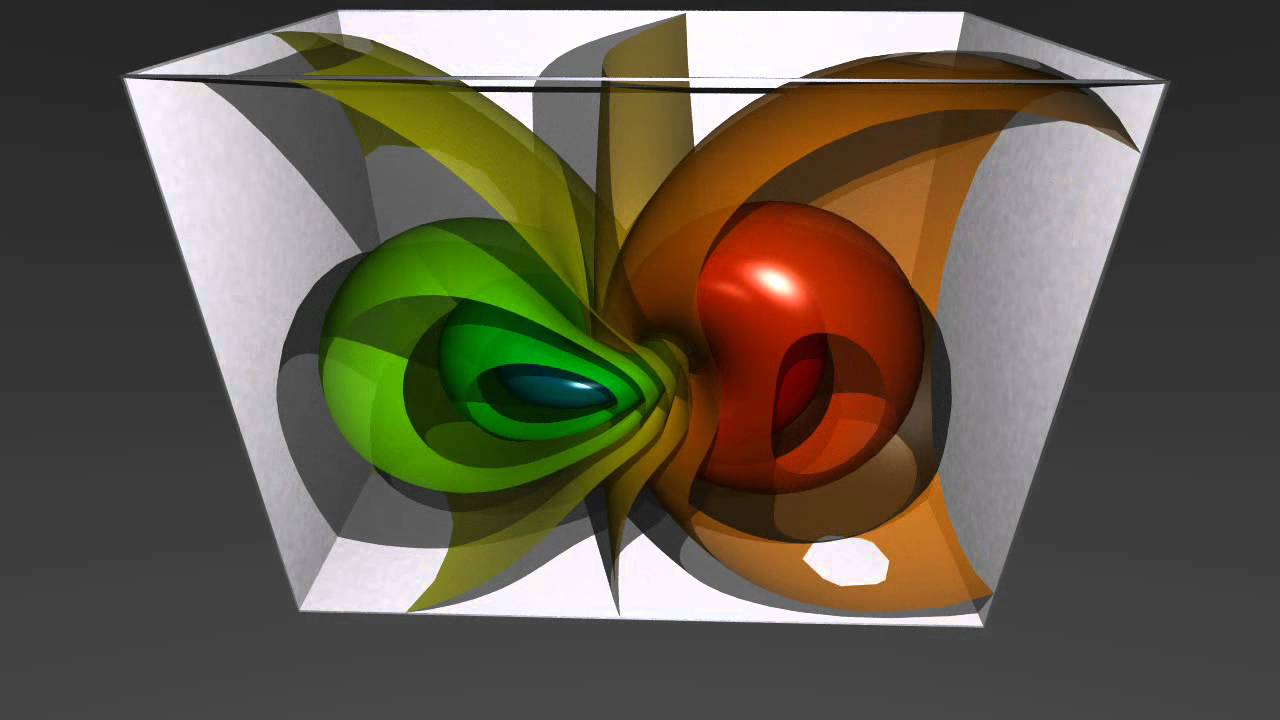The image is a highly detailed and colorful computerized graphic, depicting an abstract 3D model inside a transparent, perspective-drawn white rectangular box against a dark gray background. The main focus within the box includes a series of vibrant orbs and layers of colored planes. Inside, a central green orb houses smaller orbs and has a blue, jewel-like center. Surrounding this are layered planes that transition in color from green to yellow and orange. On the right side, an orange crescent moon-shaped layer wraps around a bowl-shaped red layer. Dominating the middle area are yellow spikes, resembling a spider. Lower down in the structure, a white polygon is cut from one of the bottom layers, adding to the complexity of this abstract modern art piece.